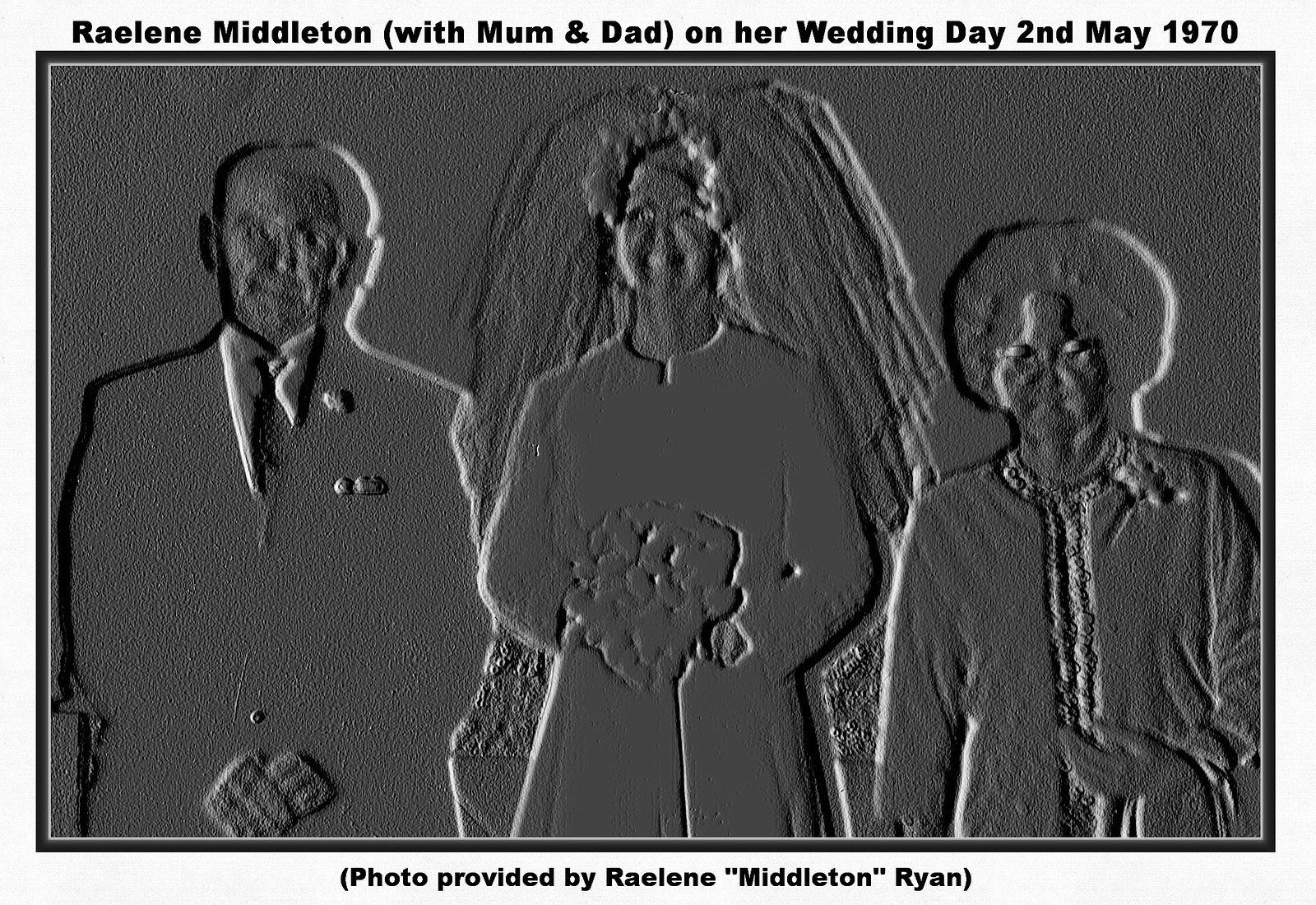The image is a highly manipulated wedding photograph rendered in shades of gray and black, resembling a photographic negative with an embossed texture. The central figure is a smiling bride in a wedding dress, holding a bouquet, with a veil trailing behind her. Flanking her on either side are her parents: an older man in a suit and tie stands to her left, and an older woman with curly hair stands to her right. The caption above the image reads, "Raylene Middleton with mom and dad on their wedding day, 2nd of May, 1970," while below it says, "Photo provided by Raylene Middleton Ryan." The image appears heavily distorted, possibly indicating an attempt at restoration. The entire photo is framed in dark gray, bordered by white with black text.